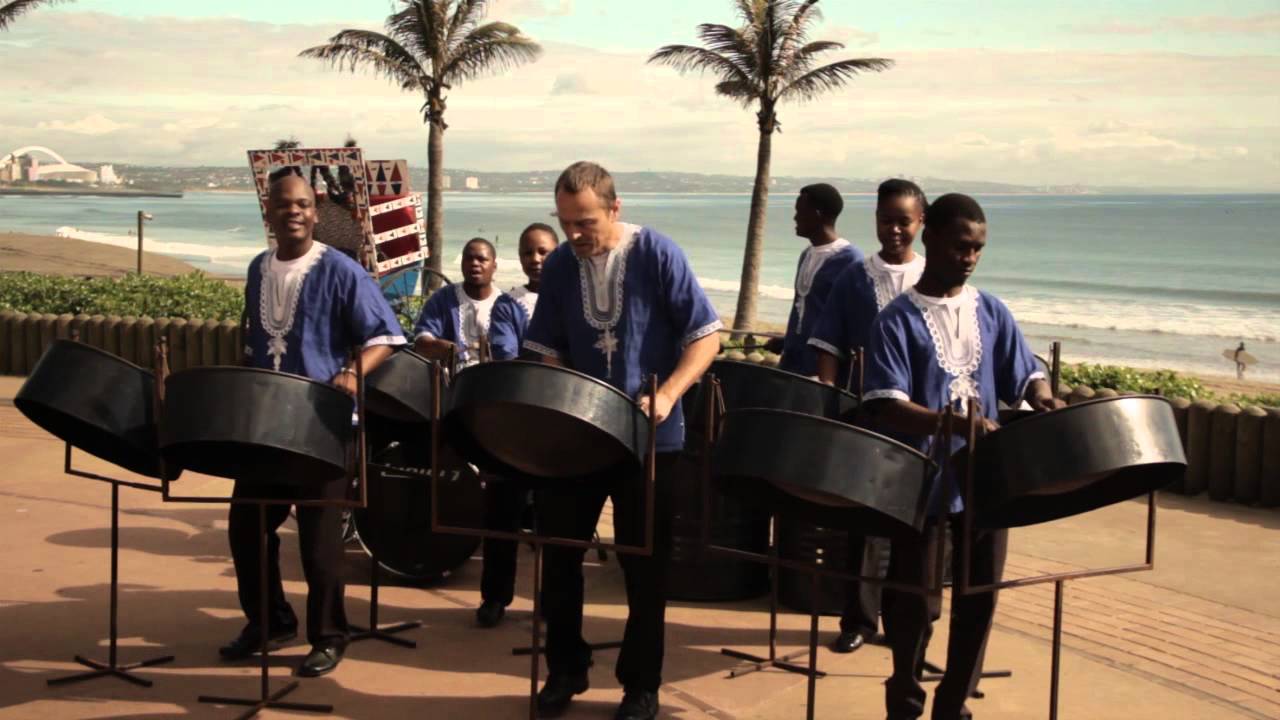A captivating beachfront scene showcases a diverse band of musicians performing on a sunlit patio. At the forefront, several members are enthusiastically playing shiny black steel drums, their melodious tunes resonating in the warm ocean breeze. In the background, faintly visible, other band members can be seen playing various instruments, including a traditional drum set. All the performers are dressed in matching, loose-fitting, short-sleeved blue shirts adorned with white fringe and lace around the collars, lending a cohesive, yet casual, look to the ensemble. Behind them, the serene expanse of the ocean stretches out, framed perfectly by the silhouettes of two tall palm trees. The patio itself is of a rich tan stucco, tinged with a dark reddish hue, and accented with brick, adding an earthy texture to the vibrant coastal setting.